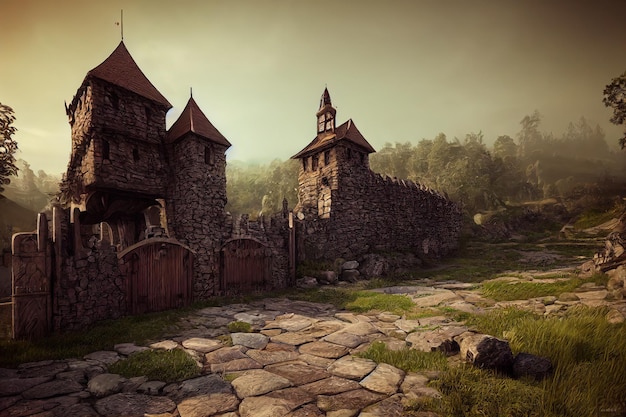The image appears to be a high-quality, photorealistic piece of digital artwork or a screenshot from a video game, possibly resembling styles found in titles like World of Warcraft. Dominating the scene is an ancient, handcrafted stone and brick structure, reminiscent of a small castle or fort, rendered in a reddish-brown hue. The stone walkway in the foreground, overgrown with grass, leads up to two sets of arched wooden gates, suggesting an entrance into a fortified property. These gates are flanked by two-story towers with sharply pointed roofs, one featuring a tall lookout turret, possibly for overseeing the property. 

The background is shrouded in a dark gray, foggy mist that lends an eerie atmosphere. Trees in various shades of green surround the structure, blending into the stone wall at the edges. The intricate details such as small windows on the towers and the varying heights of the connecting stone walls emphasize the age and craftsmanship of the scene. The overall palette of greens, browns, and grays, combined with the dark and hazy ambiance, enhances the mysterious and timeless feel of the landscape.